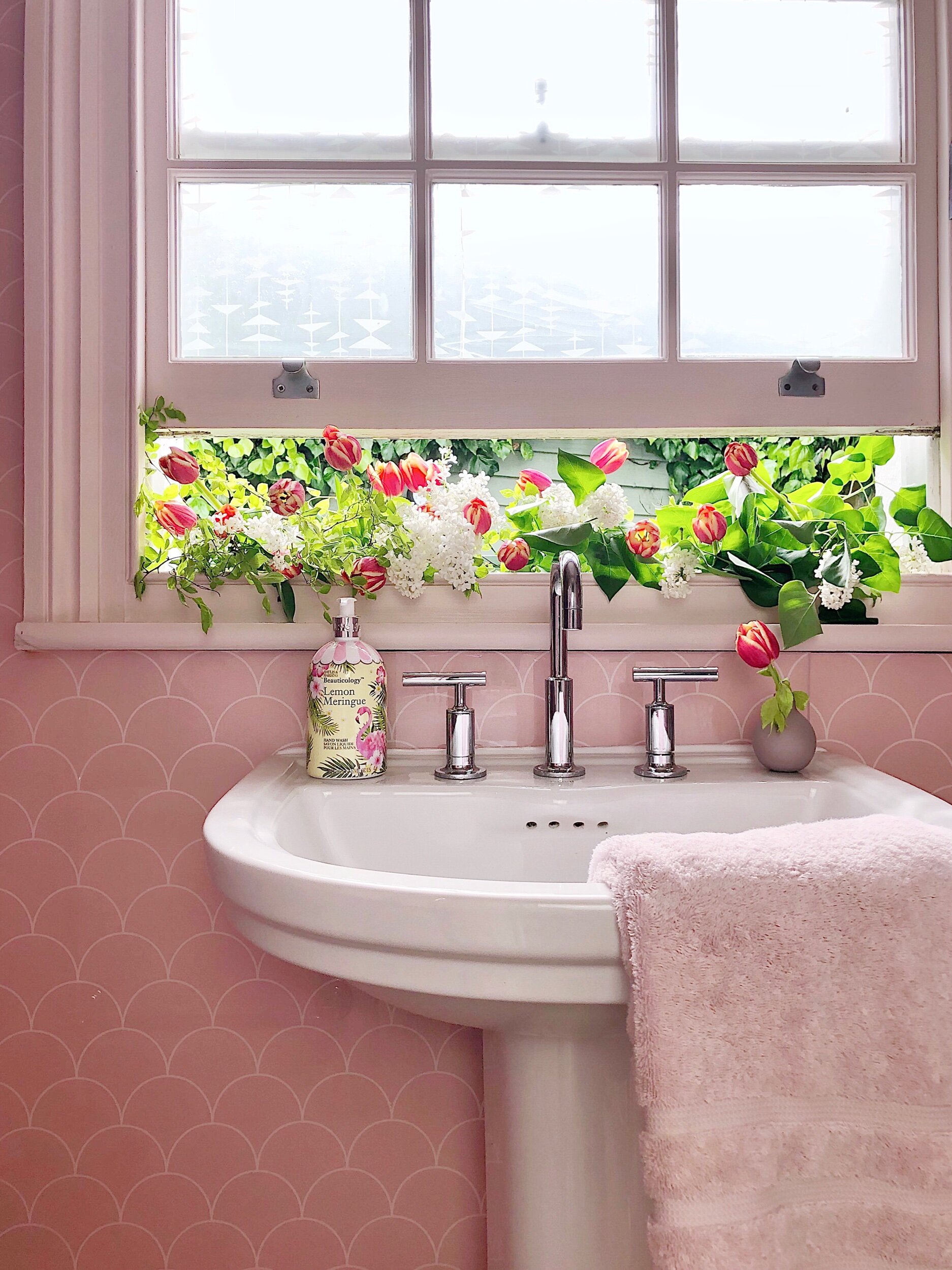This photograph captures a detailed view of a bathroom sink area, featuring an array of pink accents and floral decor. The focal point is a white ceramic pedestal sink, equipped with polished steel faucet handles characterized by their thin, straight design. A pink towel drapes off the front right side of the sink, adding a burst of color. To the left of the faucet, there’s a decorative bottle of hand soap with pink and white accents, emblazoned with the logo "Lemon Meringue" in yellow. On the right, there sits a round, gray vase holding a single flower. Above this arrangement, a window with a white frame is slightly ajar, allowing an array of flowers from outside to peek through the bottom. The backdrop is a vibrant wallpaper adorned with overlapping curved circles in varying shades of pink, reminiscent of scales. The harmonious blend of colors and elements creates a charming and serene bathroom scene.